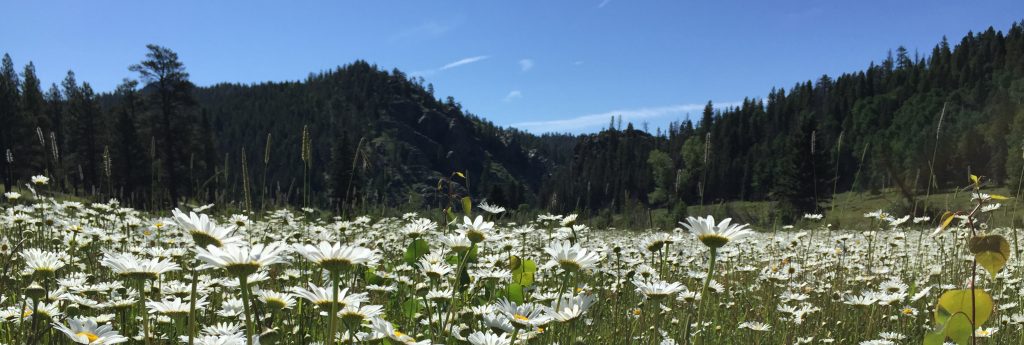The image is a horizontal rectangular photograph, taken from a low vantage point, capturing a picturesque countryside scene. It is a panoramic shot, seamlessly stitched together to form a wide strip, with minimal lines of demarcation between the sections. The foreground features a lush green field densely populated with vibrant white daisies, their yellow centers vividly contrasting against the greenery of leaves and grass. Stretching beyond the field, the background reveals gently rolling hills adorned with dense, dark green foliage, indicating a richly forested area. The time of day appears to be morning or midday, characterized by a clear, light blue sky with scarcely a cloud in sight, enhancing the serene and vibrant atmosphere of the landscape. The photograph embodies realism, offering a detailed and immersive view of the tranquil countryside scenery.